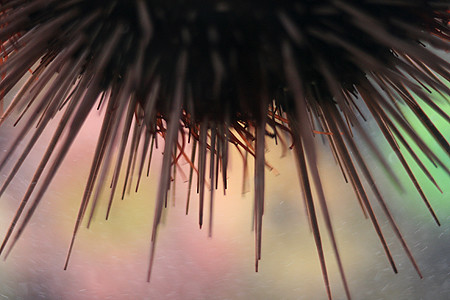The image depicts a close-up view of a vividly detailed object resembling the top of a tiki or possibly a sea urchin or spiky fruit. The centerpiece is a semicircular structure with a dark brown, fuzzy surface. Emerging from this center are numerous pale pink, sharp, long spikes of varying lengths, distributed evenly around the core. The entire scene is bathed in a hazy array of ambient lighting, showcasing pastel hues of yellows, pinks, grays, and a striking lime green to the right, evoking the warmth of a sunset. The background features blending colors of pink, yellow, and green, enhancing the impression of a warm, serene evening possibly near a beach setting. The intricate spikes and vivid colors meld together, creating a rich and inviting image that captures the essence of nature's complexity and beauty.